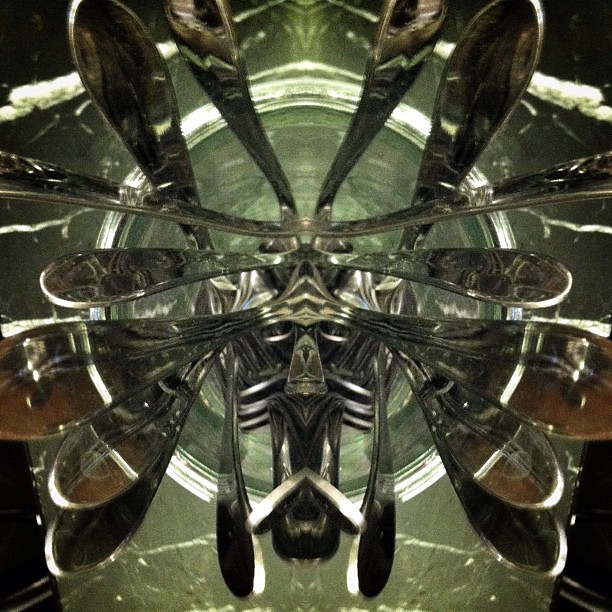The image depicts a highly symmetrical and mirrored arrangement of silverware, predominantly spoons, placed upside down in a cup or glass container. The handles and stems of the silverware crisscross intricately, creating a kaleidoscope-like effect that blends the individual pieces into a singular, cohesive pattern. This results in the appearance of a face in the center, resembling that of a monkey, with features like eyes, a triangular nose, and a thin-line mouth evident amidst the swirling silver handles. Adding to the complexity, the background shows a dual tone with a greenish hue at the top, likely from a slightly tinted glass, and a golden-brown hue at the bottom. The corners of the image fade into a darker shade, perhaps indicating a table surface or background. Collectively, the image exudes a spidery, almost surreal aesthetic, where the distinct outlines of the silverware meld together beautifully in the reflective, symmetrical display.